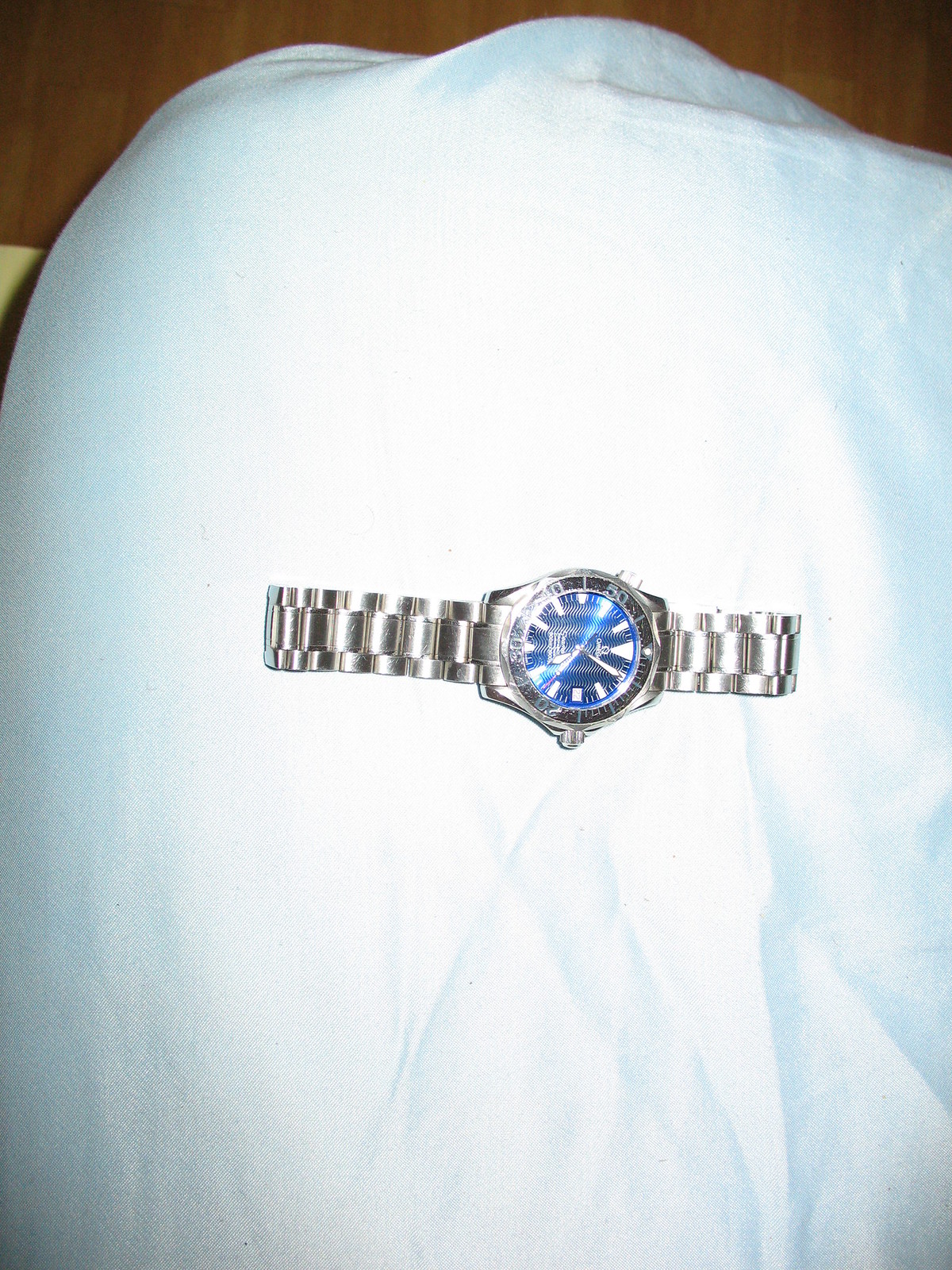In this detailed image, an Omega watch is prominently displayed against a slightly wrinkled white cloth, which appears to be either a towel or a blanket. The watch is oriented horizontally, stretching from left to right, with its band fully extended. The watch itself is a sophisticated piece, likely a high-end model such as the Seamaster, characterized by a striking deep blue face. Instead of traditional numbers, the face features sleek lines marking the hours. The watch's body and band are composed of a reflective silver metal, possibly platinum. The reflective nature of the watch is accentuated by a light source shining on it. In the background, a wooden tiled floor can be seen, adding a warm contrast to the cool tones of the watch and the cloth beneath it. The photo is captured from a top-down angle, emphasizing the elegance and detail of the timepiece.